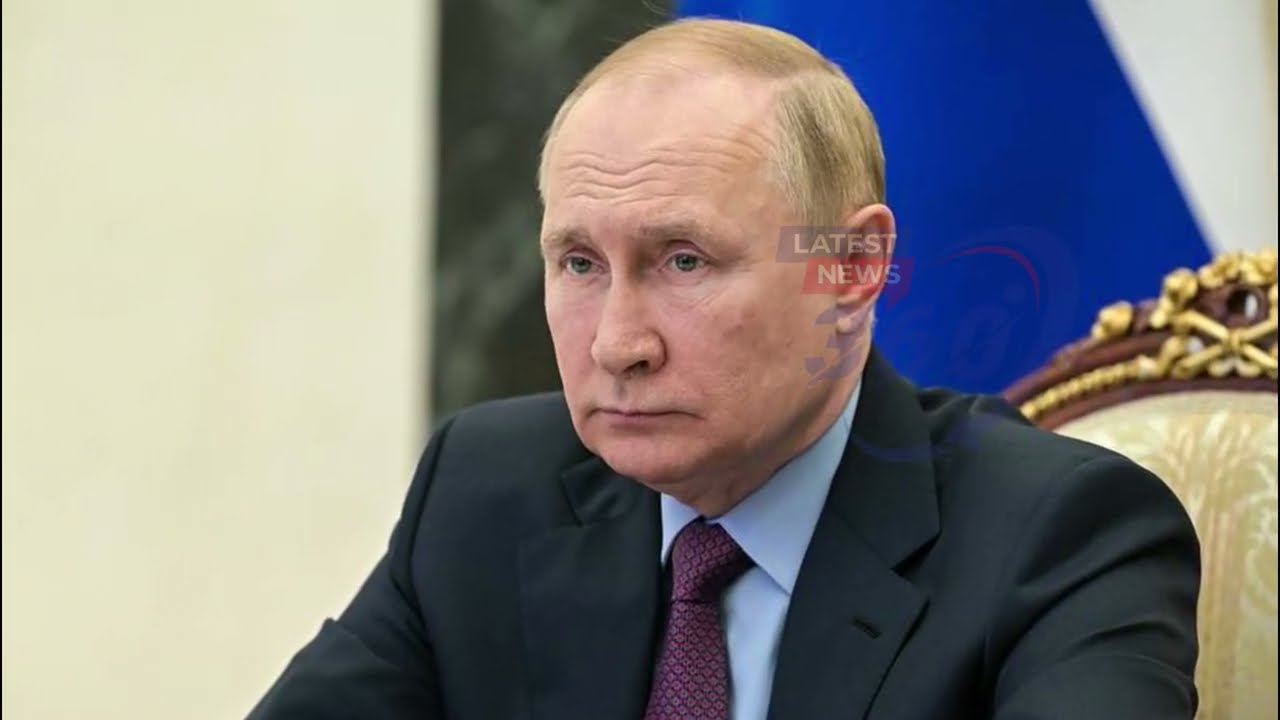The image depicts Russian President Vladimir Putin at what appears to be a paused frame from a newscast. The words "Latest News" are faintly visible, superimposed over his left ear. Putin is prominently featured in the center, seated on an elaborate chair with a brown wooden frame adorned with ornate gold decorations, including golden flowers and crisscross patterns that almost resemble a weapon. The upholstery is a light gold color. Putin sits with a stern expression, facing slightly to his left, showing a three-quarter angle of his face, shoulder, and upper chest. He has thin, light blonde hair, neatly parted and combed down the sides of his head. He is dressed in a dark suit jacket, a light blue button-up shirt, and a purple tie with a whitish diamond pattern. The background features a beige wall on the left and what appears to be a flag or drape, adding to the formal atmosphere of the setting.